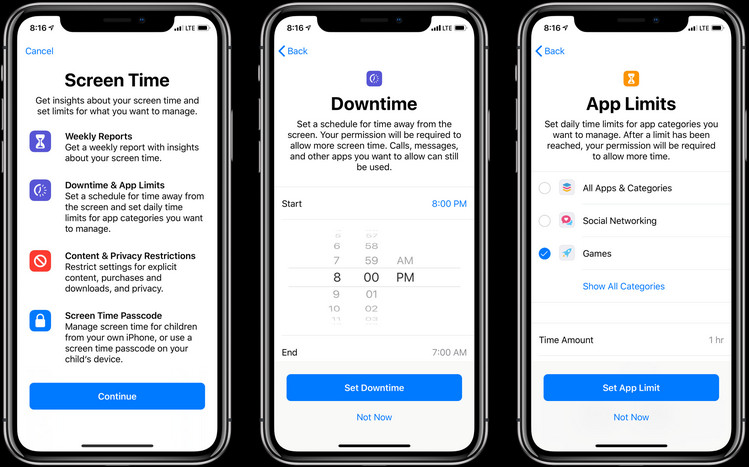In this combined image, three smartphone screenshots are presented side by side, providing a comprehensive overview of the Screen Time feature.

The first image (on the left) is divided into several sections with text descriptions:
- At the top, it reads "Screen Time" with a subtitle "Get insights about your screen time and set limits for what you want to manage."
- Below that, the section titled "Weekly Reports" states, "Get a weekly report with insights about your screen time."
- The central part showcases an icon of an hourglass set against a purple background.
- The next section is "Downtime and App Limits," which highlights the functionality to "Set a schedule for time away from the screen and set daily time limits for app categories you want to manage."
- Following that, "Content and Privacy Restrictions" talks about restricting settings for explicit content, purchases, downloads, and privacy.
- The final section at the bottom mentions "Screen Time Passcode."

In the middle image:
- The top section is labeled "Downtime" along with the instruction to "Set a schedule for time away from the screen."
- The primary visual in this screenshot features a clock set at 8 PM, indicating a scheduled downtime period.

The image on the right:
- The header "App Limits" appears at the top.
- Below this, three checkboxes are shown, with one of them labeled "Games" marked, indicating selected app categories for time management.

This detailed, visual representation provides an intuitive breakdown of the various tools and options available within the Screen Time feature, designed to help users manage and monitor their device usage efficiently.